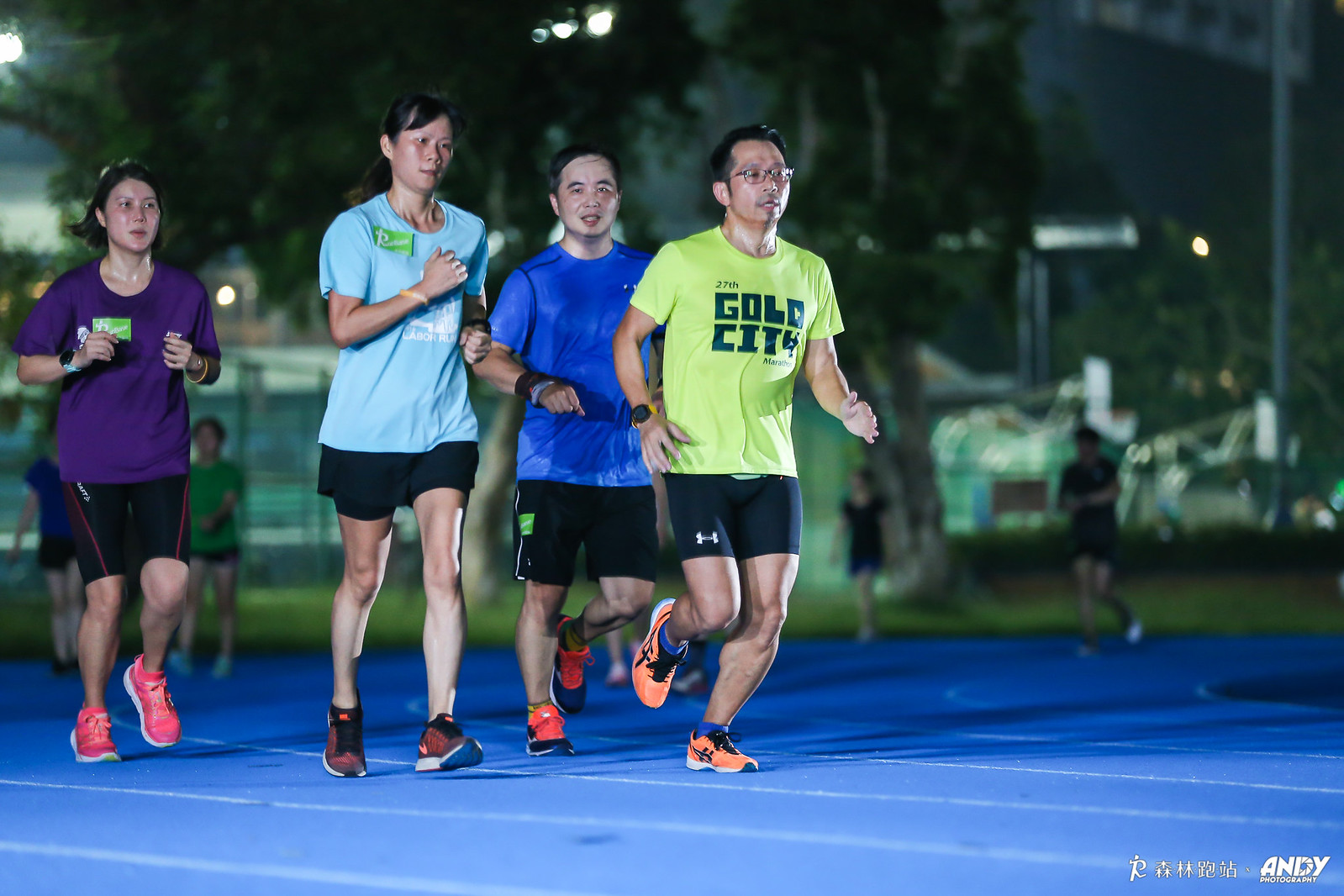Four individuals are jogging on a blue track with white lines, illuminated brightly against an outdoor nighttime backdrop. The runner in the lead sports a light green shirt with "Gold City" printed in bold black letters, along with black, tight-fitting shorts and orange Reebok shoes. This person also has black hair, glasses, and blue socks. Following closely is a man in a sweaty blue shirt and black shorts, wearing black shoes with orange shoelaces. To his left, a taller woman runs briskly, dressed in a light blue shirt with a green patch on the left shoulder, black shorts, and red shoes. Trailing the group is another woman in a purple shirt, black tight shorts, and bright pink tennis shoes. Behind them, more runners are visible but blurred, hinting at others also completing laps. The track’s surroundings, featuring some buildings, trees, and grass, frame the scene. In the bottom right corner of the image, there are decals of people running, and on the far right side, the caption "Andy Photography" is visible. All four prominently lit individuals appear to be of Asian descent.